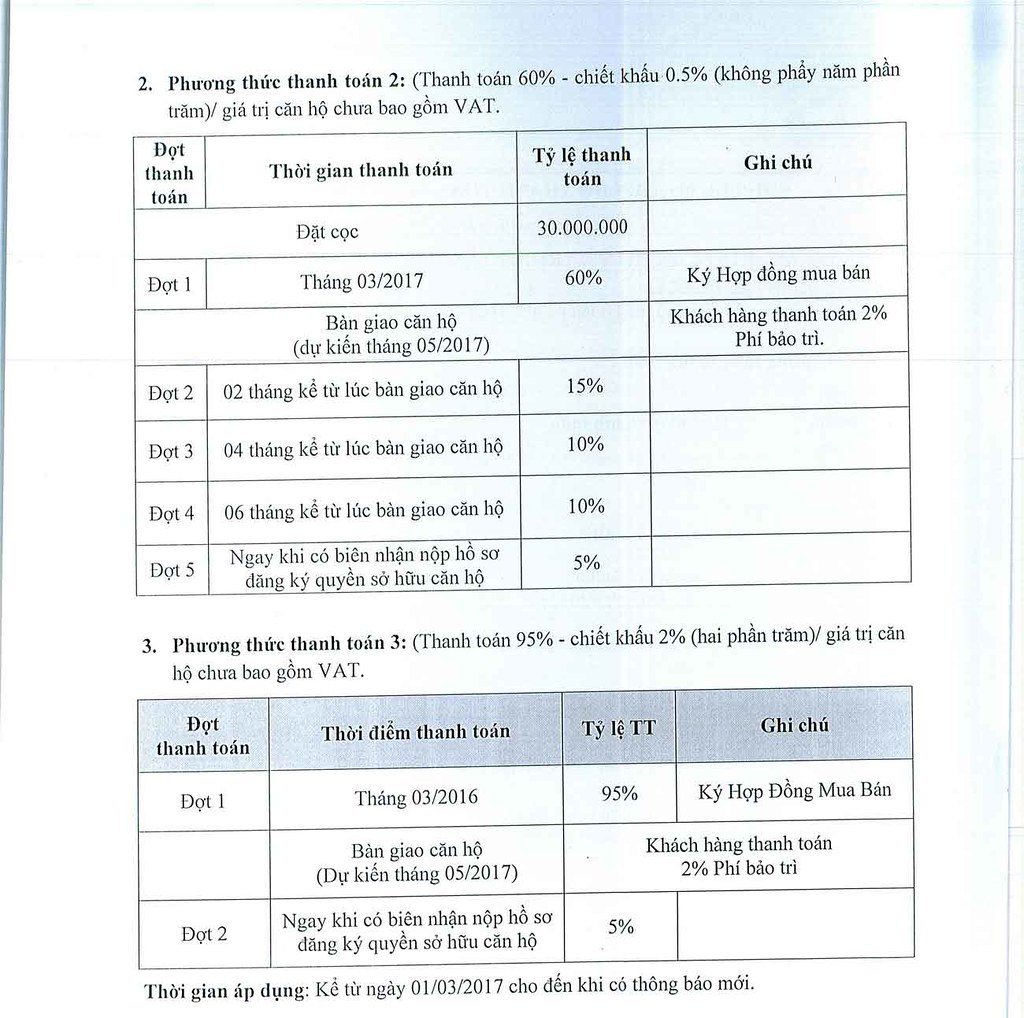The image depicts an informational sheet, likely part of a book or booklet, set against a white background and primarily written in Thai. At the top of the page, there is a bold number "2" followed by bolded Thai text providing some description, extending for a line or two. Below this text, there is a detailed table with four columns and seven rows, although a few of its cells, specifically five, are not filled in. The table’s first column seems to list days (e.g., day one, day two), with the adjacent columns containing a mixture of text and numerical data, including percentages (e.g., 60%, 15%, 10%, 5%).

Following the table, a black number "3" introduces another section in Thai with a brief unbolded line of text below it. Beneath this text, there is a second, smaller table with four columns and three rows, nearly complete except for a few entries. This table has headings at the top and lists data similar to the previous table, including days and numerical information. The page concludes with more Thai text. Numbers and percentages prominently featured include 2, 3, 30, 60%, 15%, 2%, 5%, and dates like 3/2016 and 1/3/2017.